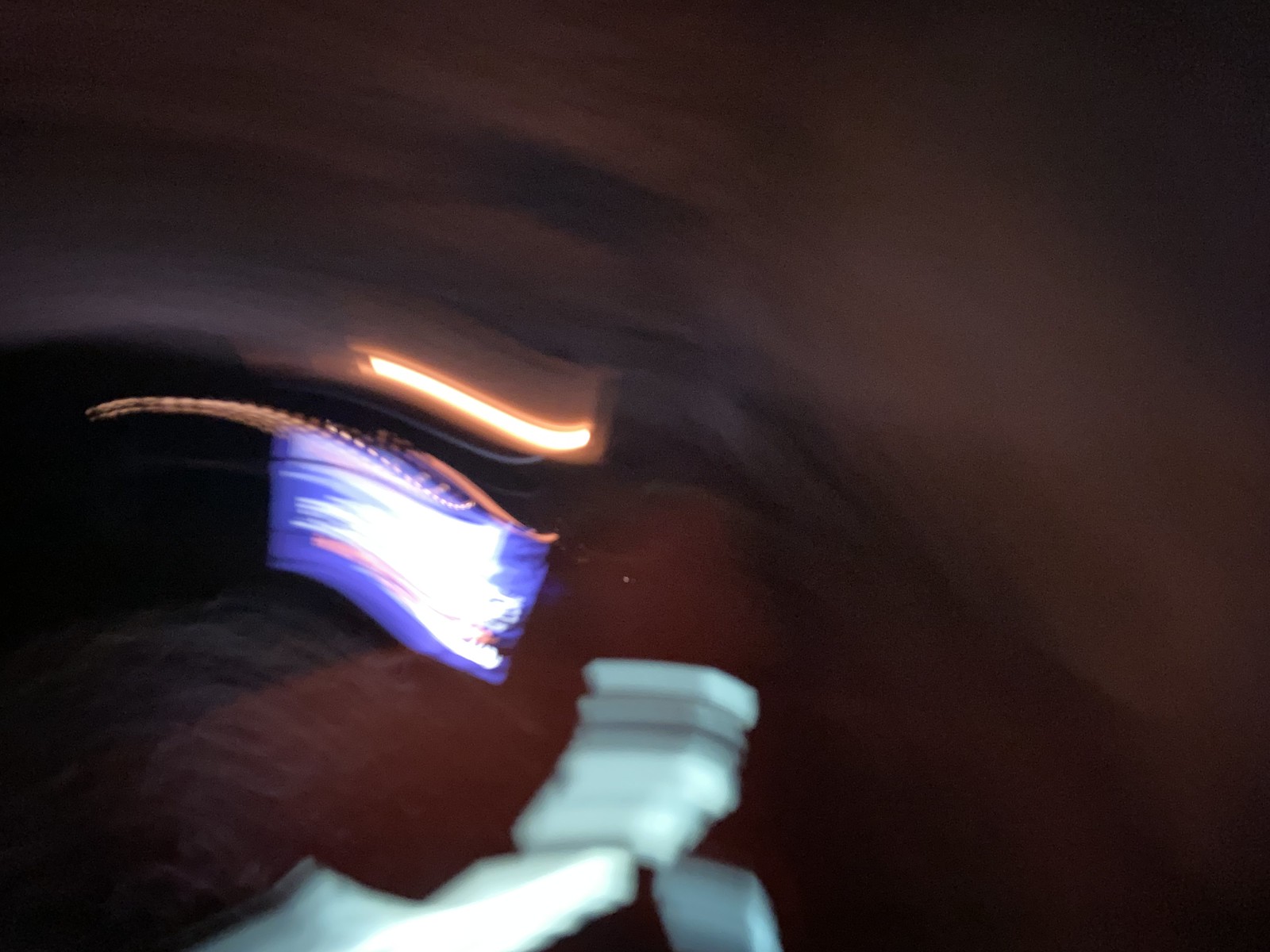A dynamic scene featuring an array of lights and colors in motion dominates the image. Amidst a nearly opaque background, a cascading series of white and gray domino-like shapes seem to tumble, suggesting rapid movement from left to right. The brightest focal point is a radiant white light embedded within a swirl of blue hues, punctuated by striking orange streaks. This vibrant light source adds depth and highlights the chaotic yet mesmerizing interplay of abstract elements.